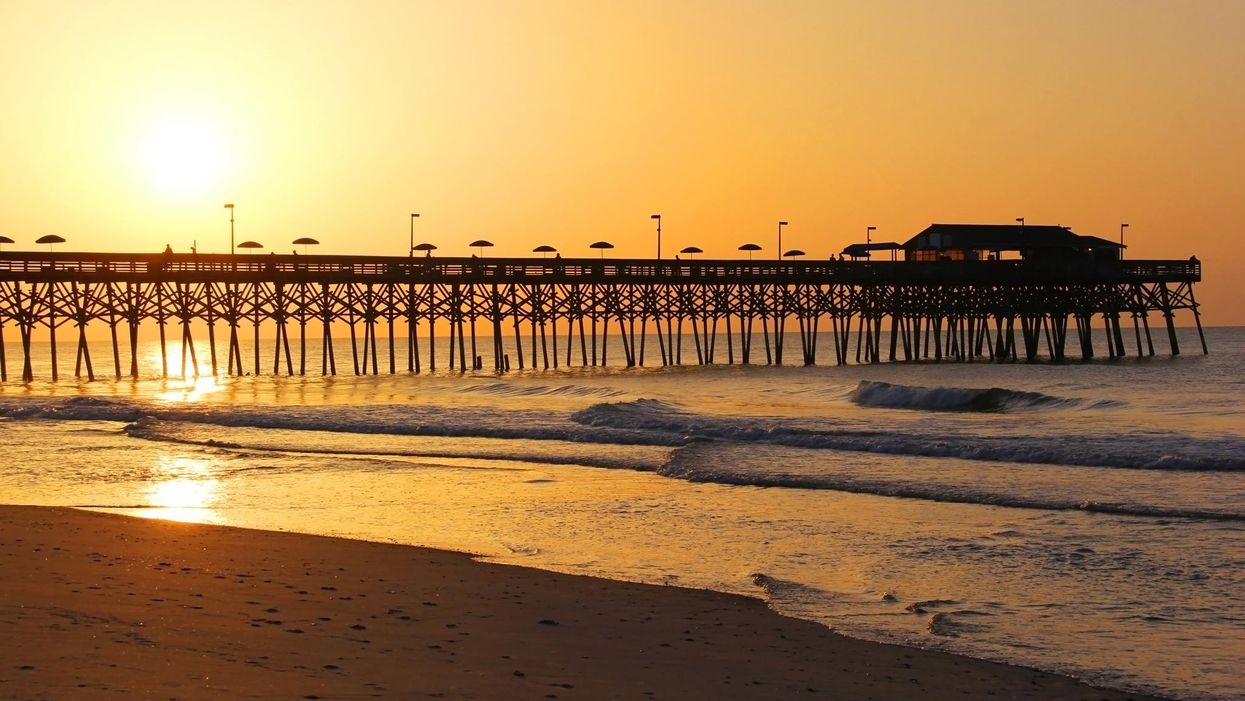The photograph captures an enchanting outdoor seaside scene during the evening. In the foreground, on the lower left corner, a beach with visible footprints extends into a tranquil ocean. A long pier, adorned with numerous umbrellas and light posts, stretches from the middle left to nearly the middle right of the image. The pier, constructed with many trusses and having a fence along its edge, leads to a structure at its end, which could be a house or an open-walled building with a roof. In the background, the sky transitions to a mesmerizing palette of yellow and orange, hinting at a setting sun whose reflection shimmers on the calm sea. Waves gently wash up on the shore, blending the serenity of the water with the peacefulness of the twilight sky.